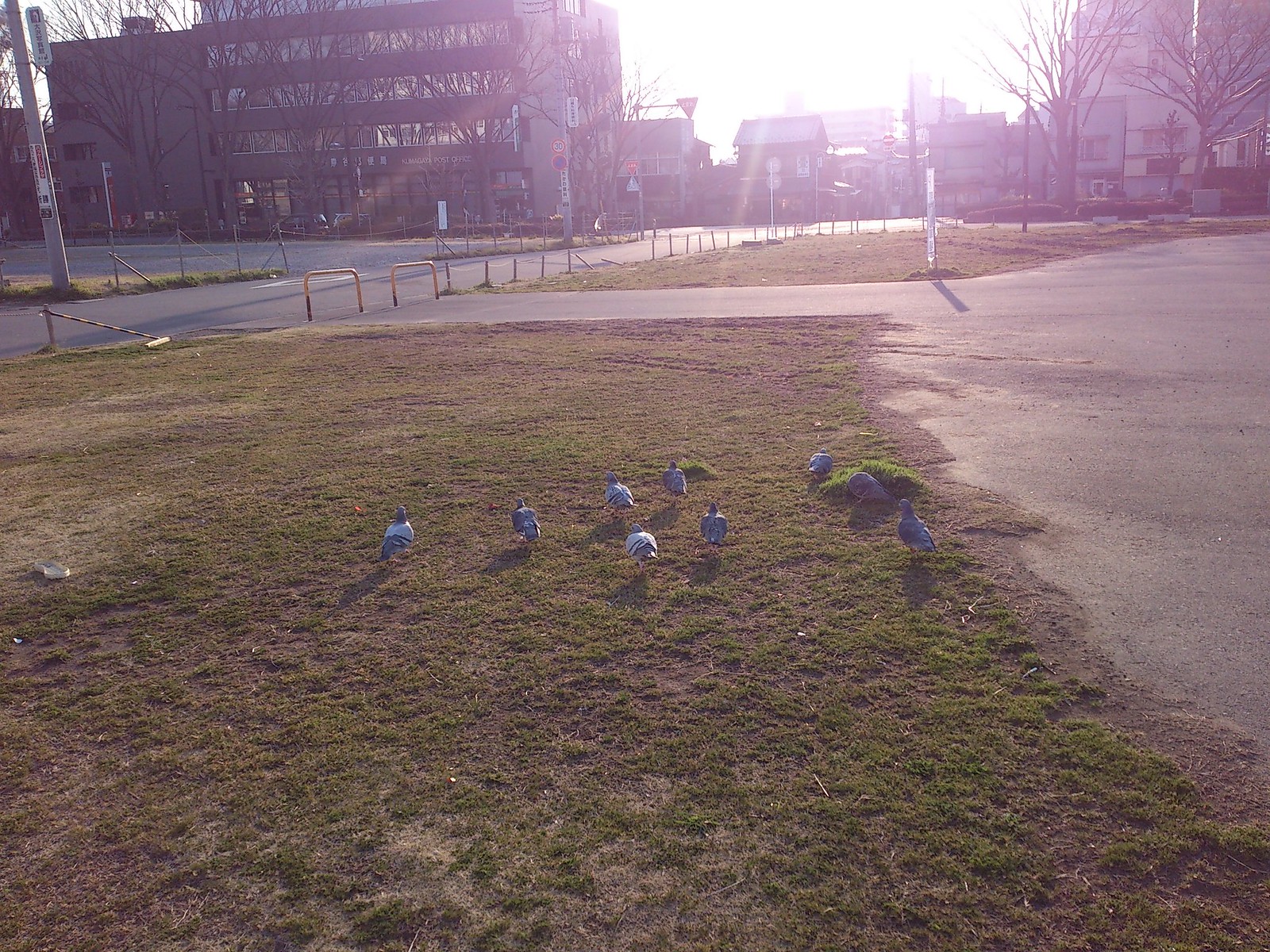The image captures an outdoor scene bathed in the warm, diffuse light of sunrise or sunset, adding a distinct purple tint and some lens flare. In the foreground, nine pigeons, predominantly grey and off-white, stand on a grass field that appears unhealthy and patchy, indicative of fall or winter. The pigeons are mostly facing away from the camera, oriented towards the sun. To the right of the pigeons, there is a paved parking lot and a road that runs across the image, with more green grass visible beyond it. The background features a variety of buildings: a prominent four-story structure on the left, several smaller buildings and homes in the middle, and another large, multi-storied building on the right. Additionally, barren brown trees are visible to the far right, hinting at seasonal change. There is also a tall silver pole with a sign on it in the top left corner, standing out against the skyline.